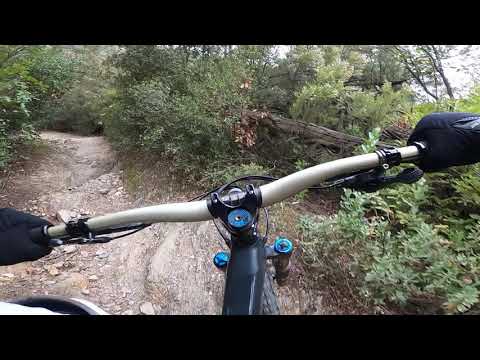This image is an exterior daylight color photograph, likely a still from a GoPro video, capturing a first-person view of someone mountain biking through a rocky, dirt trail in a wilderness setting. The scene is framed by horizontal black letterbox bars at the top and bottom. Prominently in the center, we see the silver or brass-colored handlebars of the bike, adorned with blue-topped shock absorbers, and the black-gloved hands of the cyclist gripping them. The bike itself has a black frame with blue forks. The rider is navigating a narrow, well-worn brown and gray dirt path dotted with rocks and irregularities. The path curves to the left around a large fallen log, indicating the biker's imminent left turn. Surrounding the trail, there is abundant greenery, composed of scattered green trees and dense shrubs, adding vivid color to the scene. In the upper right, the sky is visible, painted in a whitish-gray hue, suggesting an overcast day. The slight blur in the image conveys the action and movement of the ride, though the motion is not overly fast given the clarity of most details.